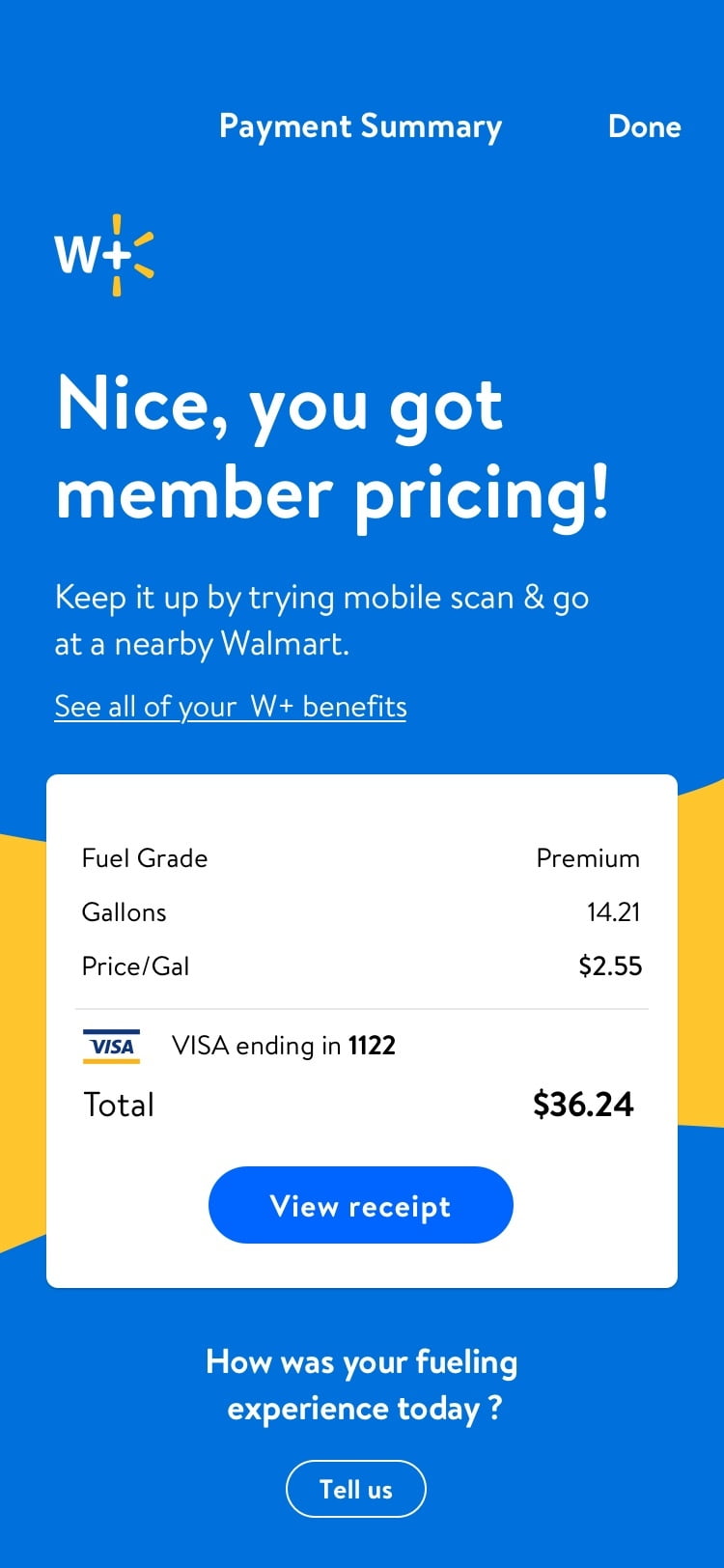This image is a screenshot of someone using the Wal-Mart shopping app, specifically within the Payment Summary section for a fuel purchase. The vertical rectangular screenshot is dominated by a deep blue color, interrupted by a wavy center line that creates a middle yellow section.

At the top right corner in white letters, it says "Payment Summary," and on the far right, "Done." Below, on the left side, is the Wal-Mart Plus logo, accented with little yellow lines around the plus sign. Further down, in large, bold white text, it states, "Nice, You Got Member Pricing," followed by smaller white text advising, "Keep It Up By Trying Mobile Scan and Go at a Nearby Wal-Mart. See all your Wal-Mart Plus benefits."

A white pop-up window in the center of the image displays transaction details. On the left side, it lists "Fuel Grade," "Gallons," and "Price/Gallon." The right side provides the corresponding information: "Premium" fuel, cost of "$14.21" for the fuel, and a price of "$2.55 per gallon." Below a gray line at the bottom of the pop-up, a Visa logo appears with the text "Visa Ending in 1122." The total payment amount is shown as "$36.24." Beneath this, a prominent blue oval button with "View Receipt" in white letters invites action.

At the bottom of the screenshot, in bold white lettering against the remaining blue background, the question "How Was Your Fueling Experience Today?" is posed. Below, another blue oval button outlined in white, with the text "Tell Us" in white letters, offers a way to provide feedback.